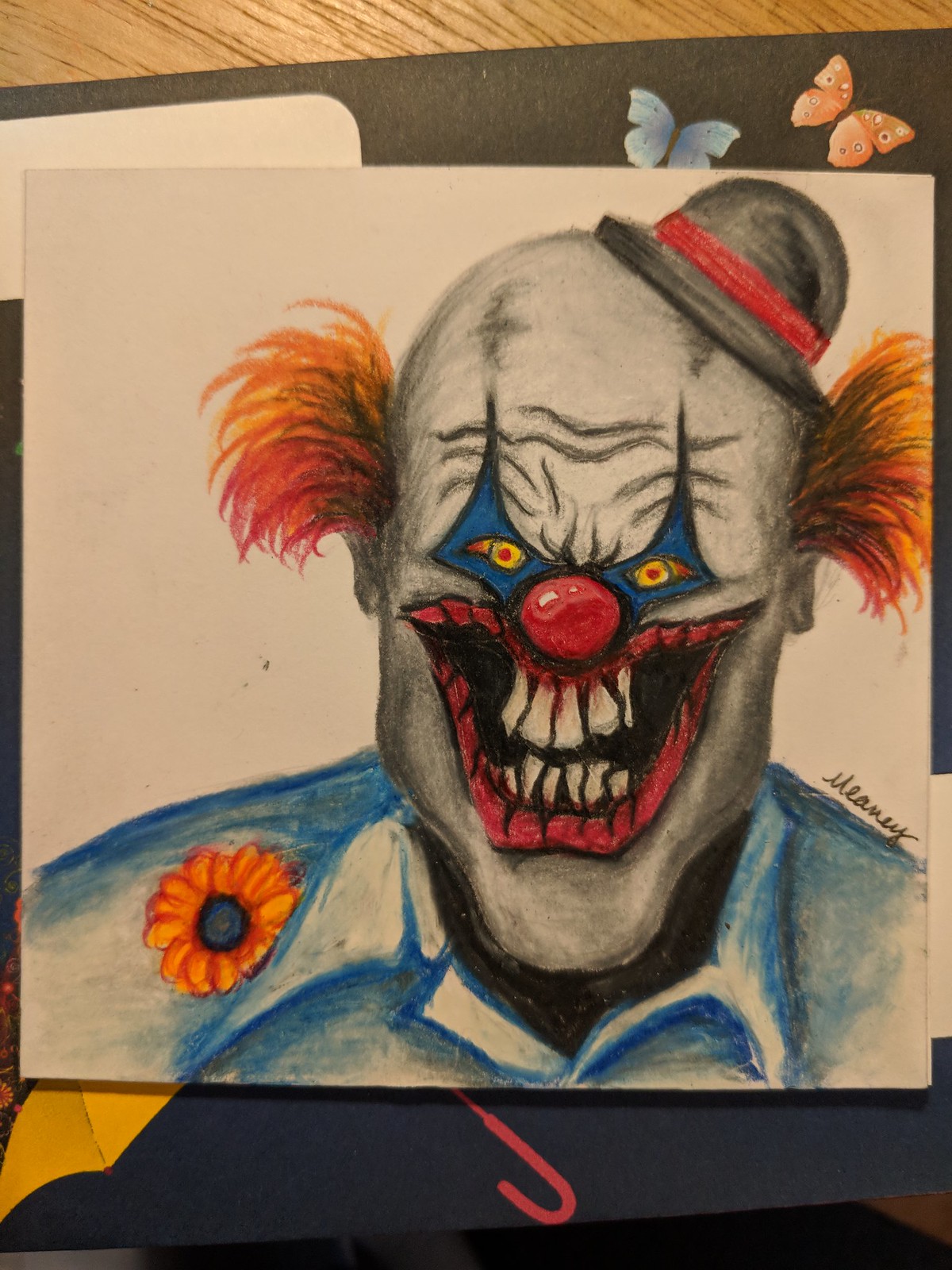This detailed drawing depicts a ghastly clown figure centered on a white background, intricately rendered with colored pencils. The clown's white, deeply wrinkled face is contrasted by ominous black lines across his forehead and eerie blue triangles framing his sinister yellow eyes. Perched atop his head is a tiny black derby hat adorned with a red ribbon, and orange tufts of hair jut out from either side. His expression is menacing, featuring a large, red-rimmed mouth exposing skeletal teeth—five on the top and six on the bottom—set against a dark, hollow background. The clown's bright red nose enhances his disturbing visage. He sports a light blue shirt, accented by an orange flower on his right shoulder. The entire image is surrounded by a border that hints at another picture beneath it, showing fragments of an umbrella and displaying blue and orange butterflies on a dark section of the background. The piece is signed "MEANEY" just above the clown’s right shoulder.